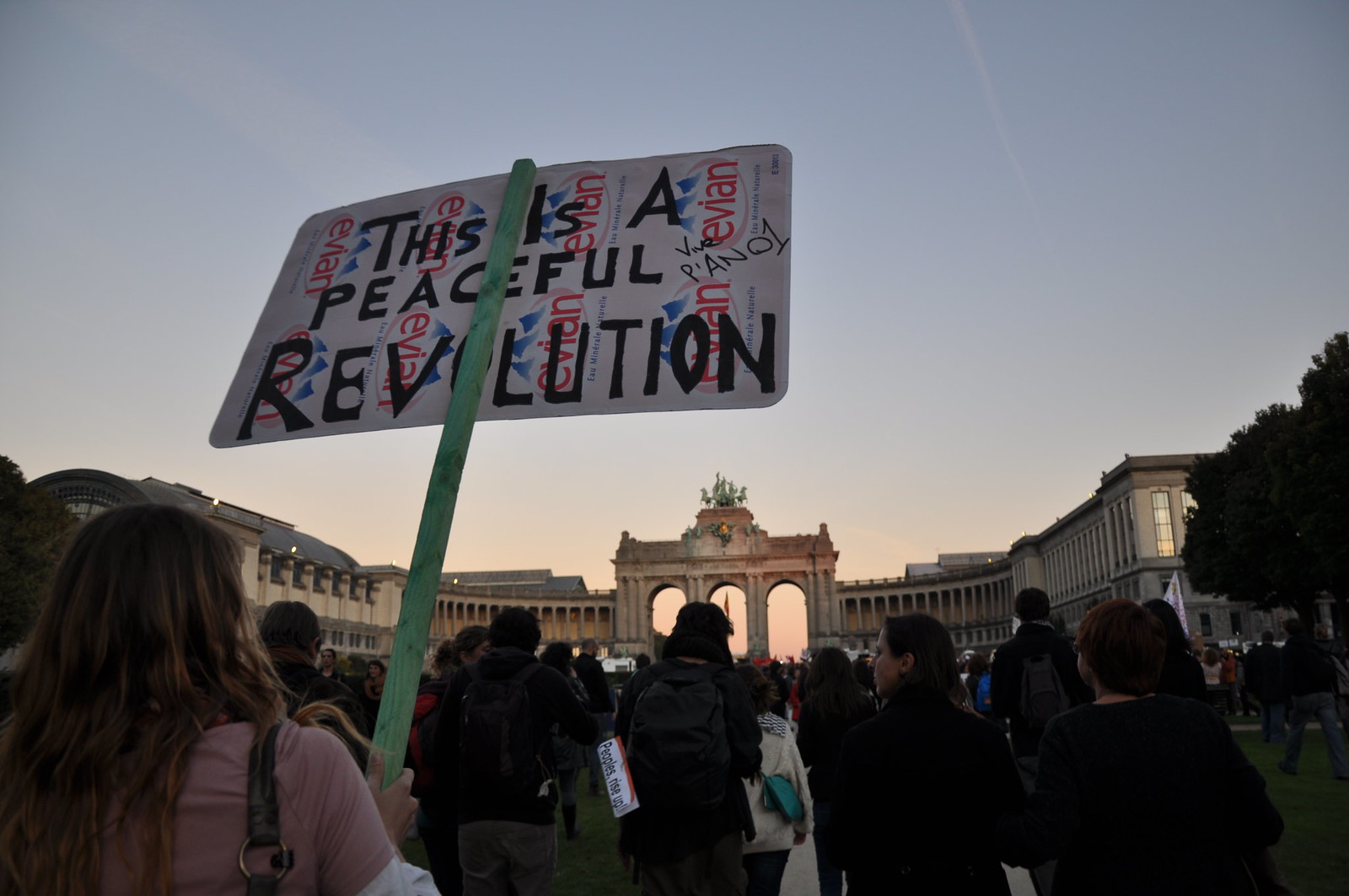The photograph captures a twilight protest at the iconic Brandenburg Gate in Berlin. The scene, set against a backdrop of large, classic buildings with columns, is bustling with hundreds of demonstrators, many of whom are students dressed largely in dark clothing. The sky is adorned with a gradient of blue transitioning to a reddish hue, suggesting a setting sun. Foregrounded in the image, on the bottom left, stands a woman with brownish hair donning a tan t-shirt over a white shirt, holding a makeshift sign fashioned from an Evian water carton. The sign, mounted on a wooden stick, prominently reads, "This is a peaceful revolution," with additional Evian logos visible on the back. The atmosphere remains calm and orderly, reinforcing the peaceful nature of the protest as attendees walk towards the monumental gate with its central arch crowned by horse statues. Grass and trees further frame the serene evening scene.